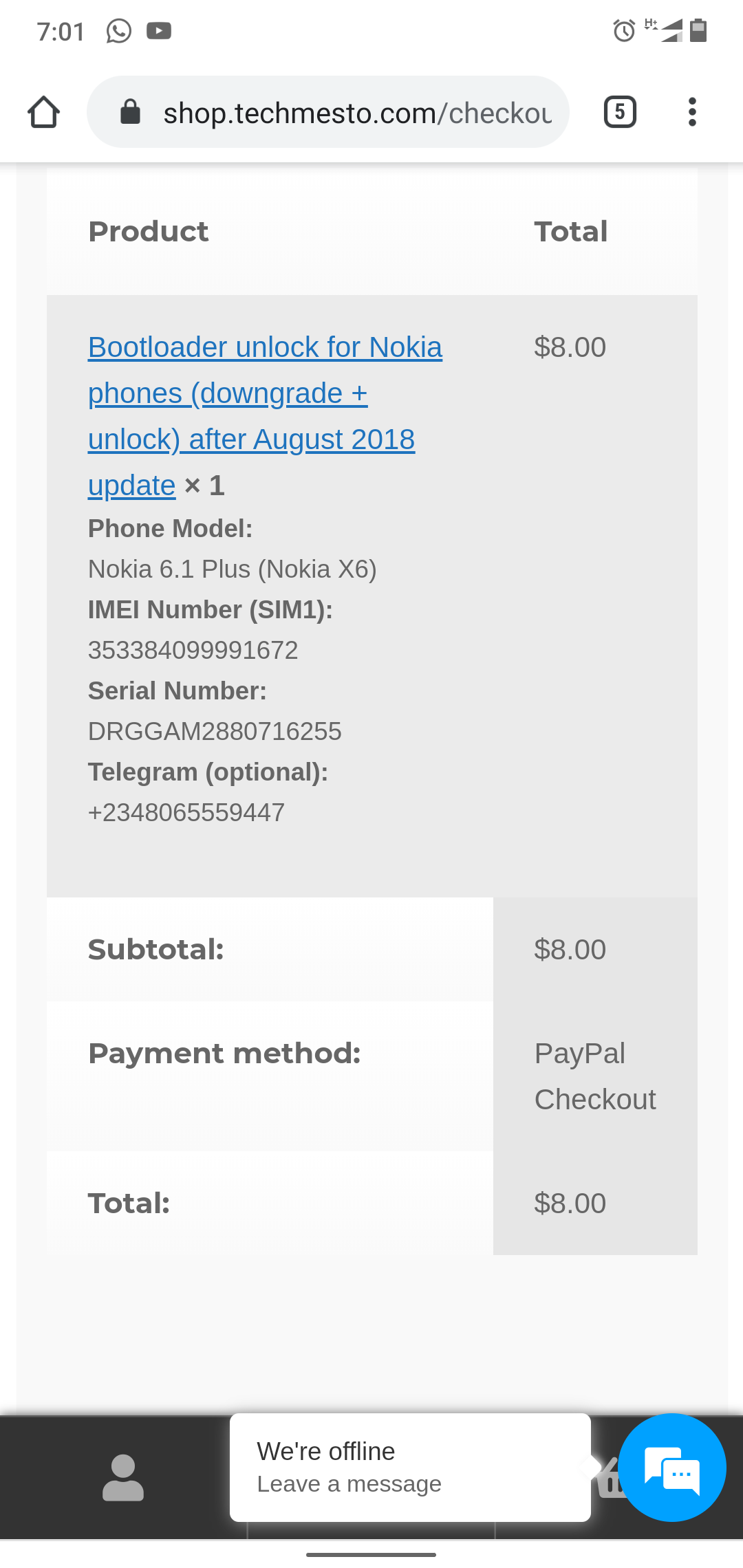A detailed screenshot from a smartphone displays comprehensive information about a transaction on shop.techmesto.com. The time, prominently shown in the upper right corner, is 7:01, while the battery icon on the left indicates about 50% charge. An active alarm icon is also visible. The search bar highlights a recent query for "shop.techmesto.com," exploring purchase options.

Just below the search bar, a clickable menu represented by three dots promises additional information. Moving further down, a table appears with "Product" listed on the left and "Total" on the right. The product details, highlighted in gray, describe "Bootloader Unlocked for Nokia Phones," specifically for models Nokia 6.1 Plus (Nokia X6) with support for downgrades and unlocks after August 2018 updates. Information specific to the phone, such as the IMEI number and serial number, is included, with contact details via Telegram also available.

Details on the right column present the pricing structure: the product subtotal is stated as $8.00, with PayPal designated as the payment method, culminating in a total charge of $8.00. A note underneath mentions that the service is currently offline but encourages leaving a message for future assistance.